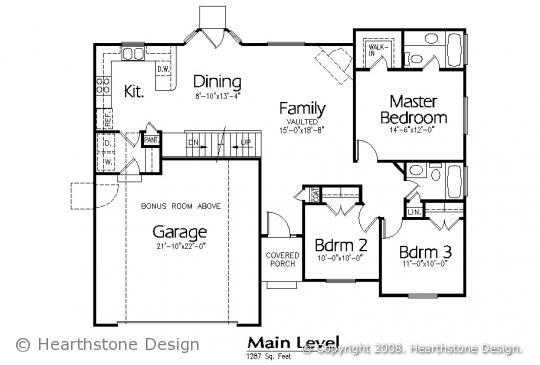This black and white image depicts a detailed blueprint of a home, showcasing various sections with precise measurements. The layout includes distinct areas such as a dining area, a family room, a master bedroom, a garage, and bedrooms labeled as Bedroom 2 and Bedroom 3. Each section is clearly annotated with dimensions. Additionally, the blueprint features a kitchen layout. In the lower left-hand corner, the text reads, "Hearthstone Design, main level, 1287 square feet, copyright 2008, Hearthstone Design."